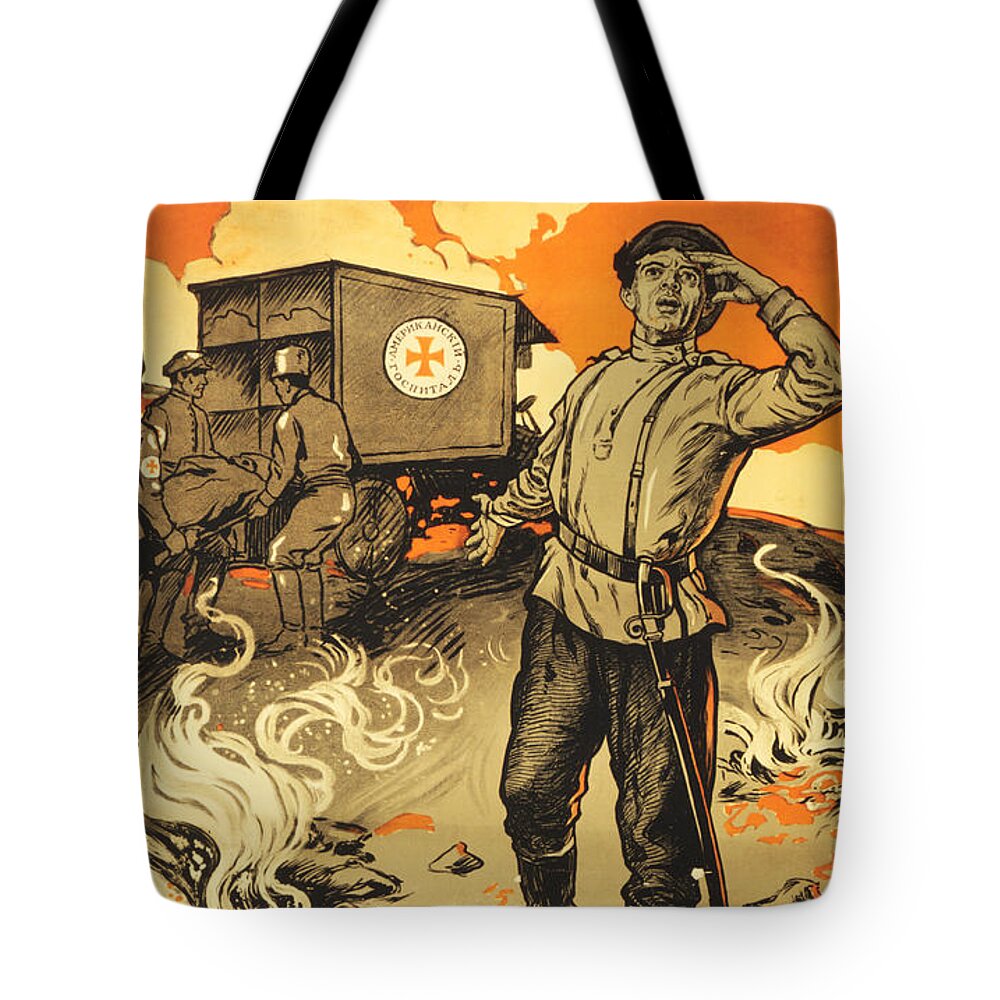This is a detailed cartoon illustration printed on a tan-colored tote bag with black straps, though the top of the straps is not visible in the image. The artwork portrays a distressing battlefield scene, likely set during World War I. At the forefront, a soldier dressed in dark pants, a light-colored shirt, and a black belt with a sword hangs wearily with his left hand raised to his forehead, looking off into the distance. The background is chaotic with fire and thick smoke filling the orange sky, enhancing the sense of turmoil. Two soldiers, clad in brown uniforms, are seen behind the main figure, loading a body into an orange-cross-marked truck, indicating medical or military evacuation. The scene encapsulates the harsh reality of war, further emphasized by the flames and artillery equipment scattered around.